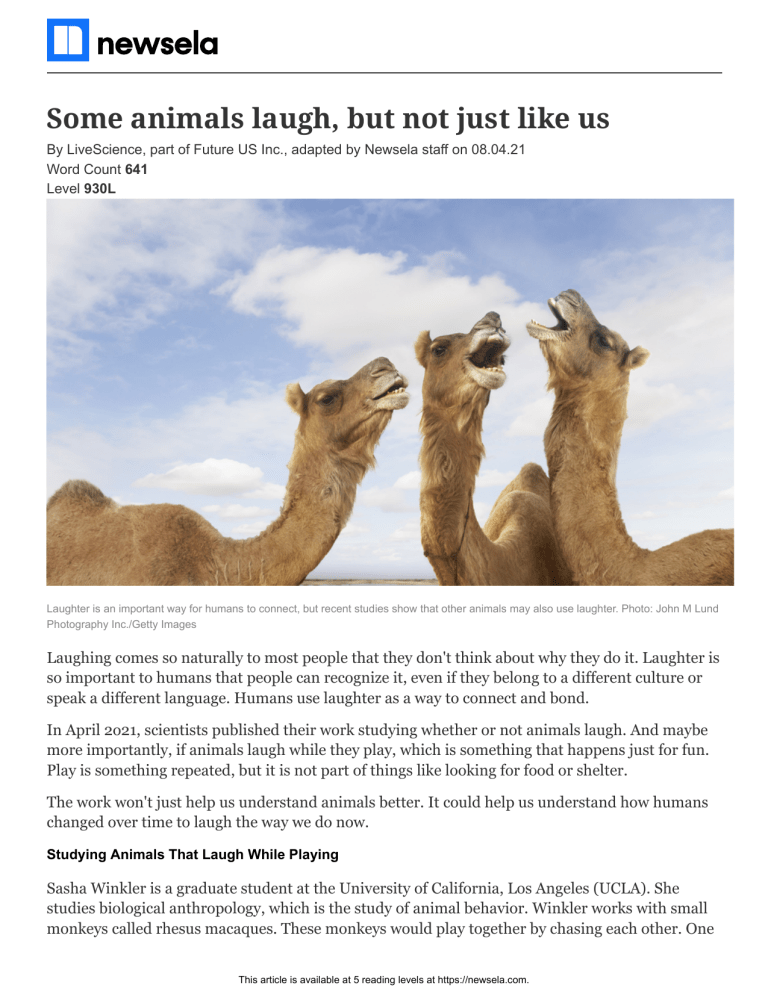This image is from a news article featured on the website Newsela. In the top left corner of the image, the Newsela logo is displayed, consisting of the word "Newsela" and an icon to its left. The icon includes a blue square with a white square inside it, featuring a blue line running through the middle, and its top right corner is rounded. The article is titled "Some Animals Laugh, But Not Just Like Us" and is credited to Live Science, part of Future U.S. Incorporated, adapted by Newsela staff on October 4, 2021. The article contains 641 words and is designated at reading level 930L. The accompanying picture shows three camels with their mouths open, appearing as if they are laughing.